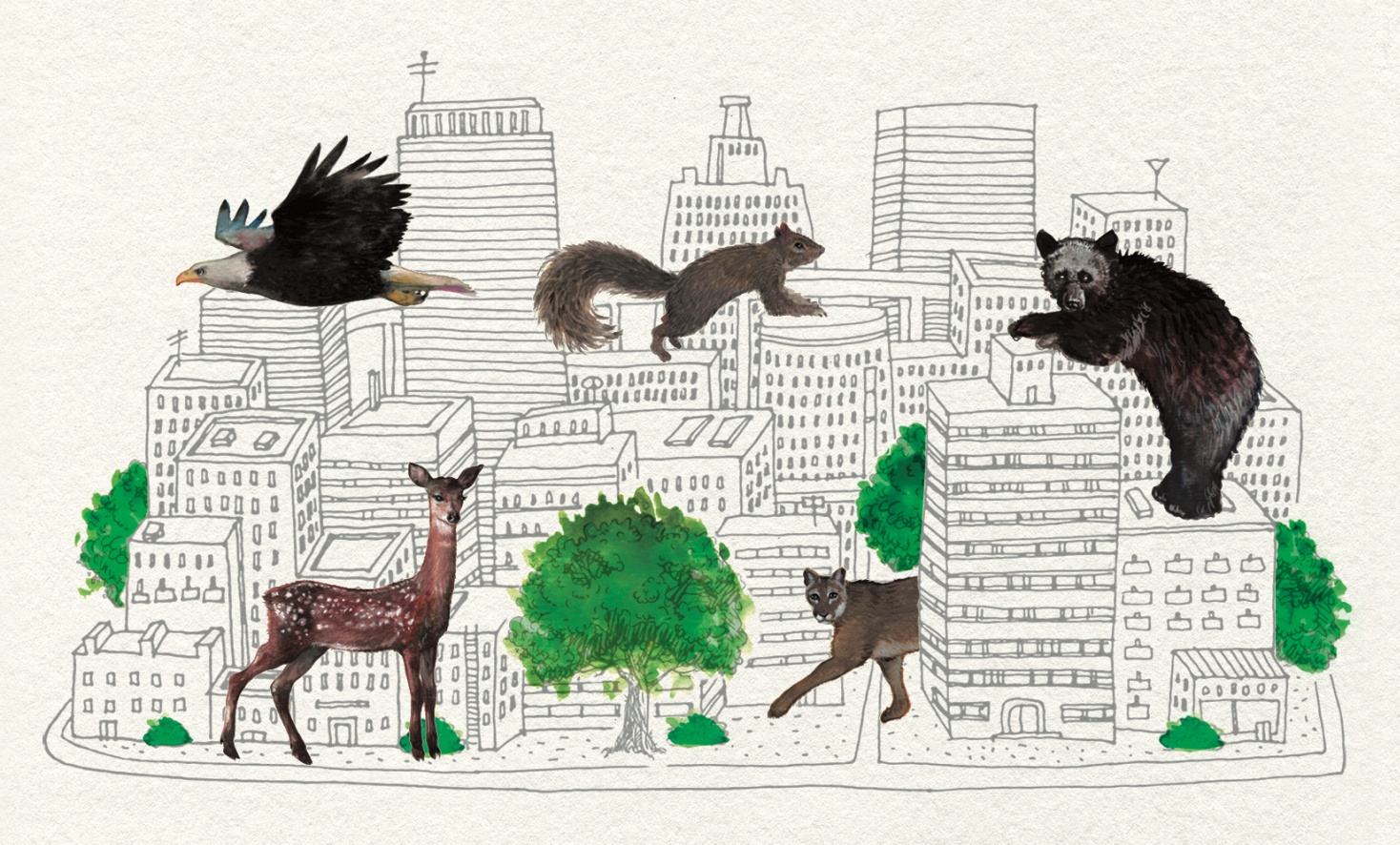The whimsical cityscape drawing, set against an off-white background, intricately details a collection of buildings rendered in black and white pencil, ranging from quaint two-story structures to imposing high-rises. Scattered amidst the monochrome architecture, vivid green trees and bushes add splashes of color, their foliage appearing life-like in bright green hues, while their trunks remain sketched in pen or pencil. This city scene becomes even more engaging with the presence of giant, realistically colored animals that dominate the cityscape. A massive black bear perches on a six-story building, clutching a taller ten-story structure for balance, gazing down at the viewer. Nearby, a large squirrel, also centrally located, uses a round structure for its front paws and a lower square building for its back paws, seemingly mid-action and looking to the right. An eagle soars gracefully over the buildings to the left, its wings spread wide. Below, a towering deer stands to the bottom left, projecting a mix of curiosity and apprehension as it gazes out from the scene. Completing the whimsical menagerie, a wildcat, possibly a bobcat or mountain lion, emerges from behind a building on the bottom right, with only its torso and head visible, poised with its feet on the pavement. Each animal, painted with lifelike vibrancy, contrasts starkly with the grayscale city, adding a fantastical element to the urban tableau.